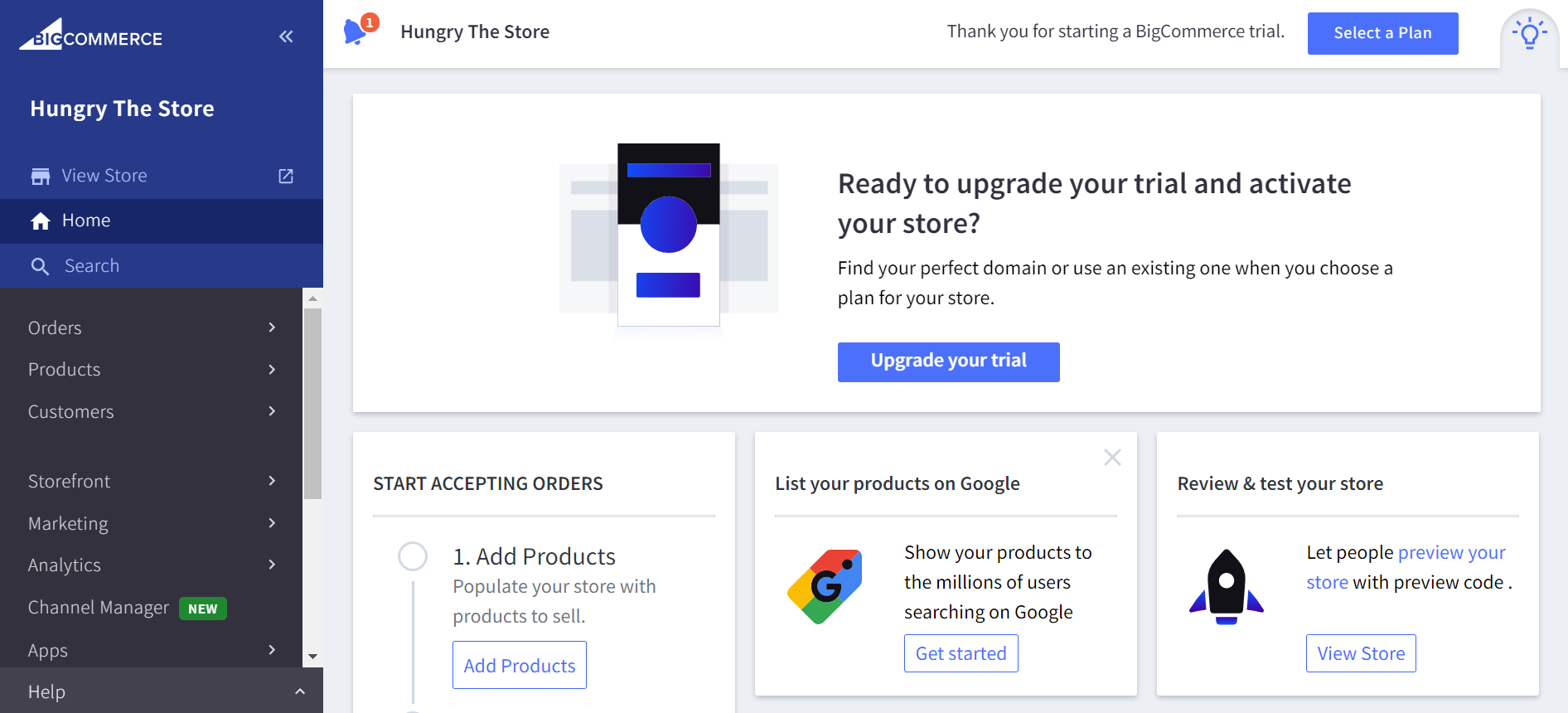This is a detailed screenshot of a website, likely an e-commerce platform. On the left side of the image, there is a blue square box with white text and icons. Prominently displayed is a white triangle with the word "Big" in blue text in front of it, followed by the words "Commerce" in bold white text. Below, there are options for "View Store" and "Home," with "Home" highlighted in dark blue, and a "Search" option underneath that.

Adjacent to this, we see a vertically aligned menu on a dark background with white text. The menu items are: "Orders," "Products," "Customers," "Storefront," "Marketing," "Analytics," "Channel Manager," and a blue button labeled "New Apps." At the very bottom of this menu, there is a dark gray banner with the word "Help."

In the upper-right section, a white banner displays "Hungry The Store" along with the message "Thank you for starting a BigCommerce trial." To the right of this text, there is a blue action button that reads "Select a Plan."